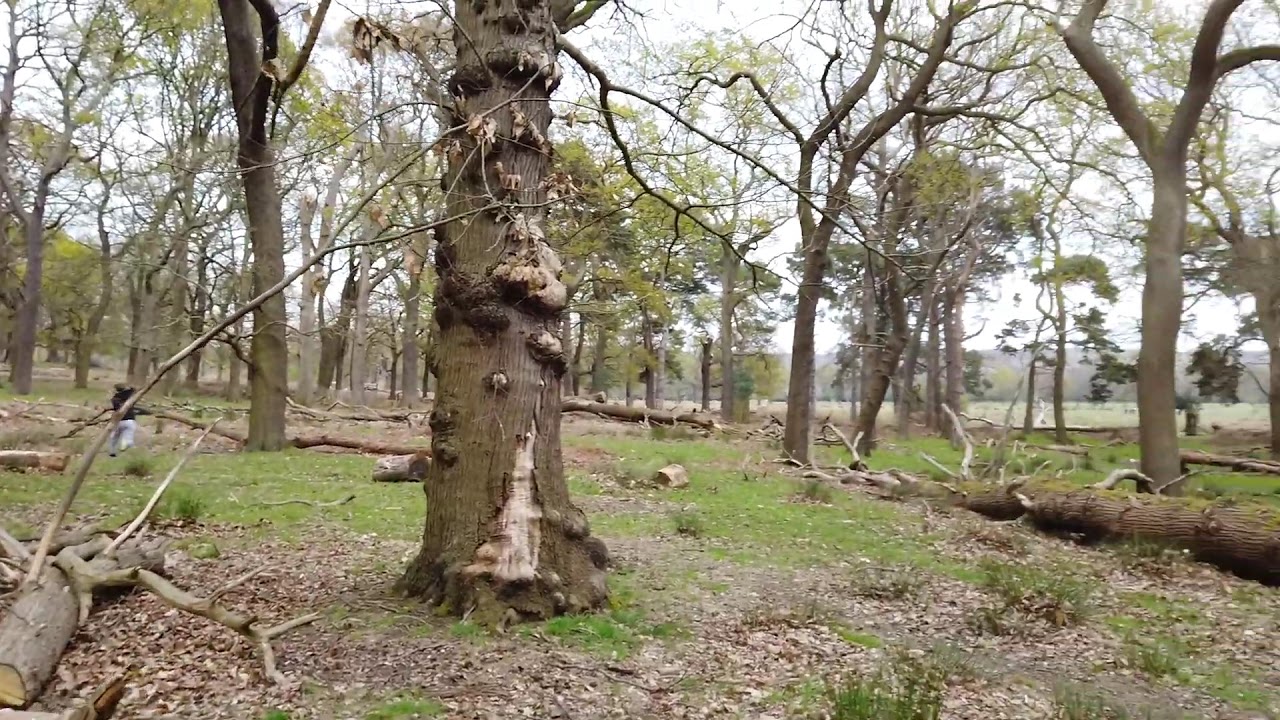In this color photograph with a landscape orientation, we see a slightly elevated view, possibly taken by a drone, capturing a lightly wooded area near a body of water, such as a river or pond, visible halfway down the image on the right side. Dominating the scene is a large, gnarly tree situated slightly left of center. This tree has a thick brown trunk adorned with numerous round, bulbous growths, possibly mushrooms or signs of disease, making it the main focal point of the image. Surrounding this central tree are various other standing and fallen trees, with some cut branches scattered on the ground, suggesting recent activity in the area. To the left, a man wearing a dark top and light pants is partially visible behind a fallen tree, perhaps engaged in cleaning up or cutting down trees. The scene conveys a sense of realism and representationalism, framed under a grey sky, with hints of autumn as some leaves have begun to fall. The photograph captures both the intricate details of the main tree and the broader natural setting, creating a striking and detailed portrayal of this woodland area.